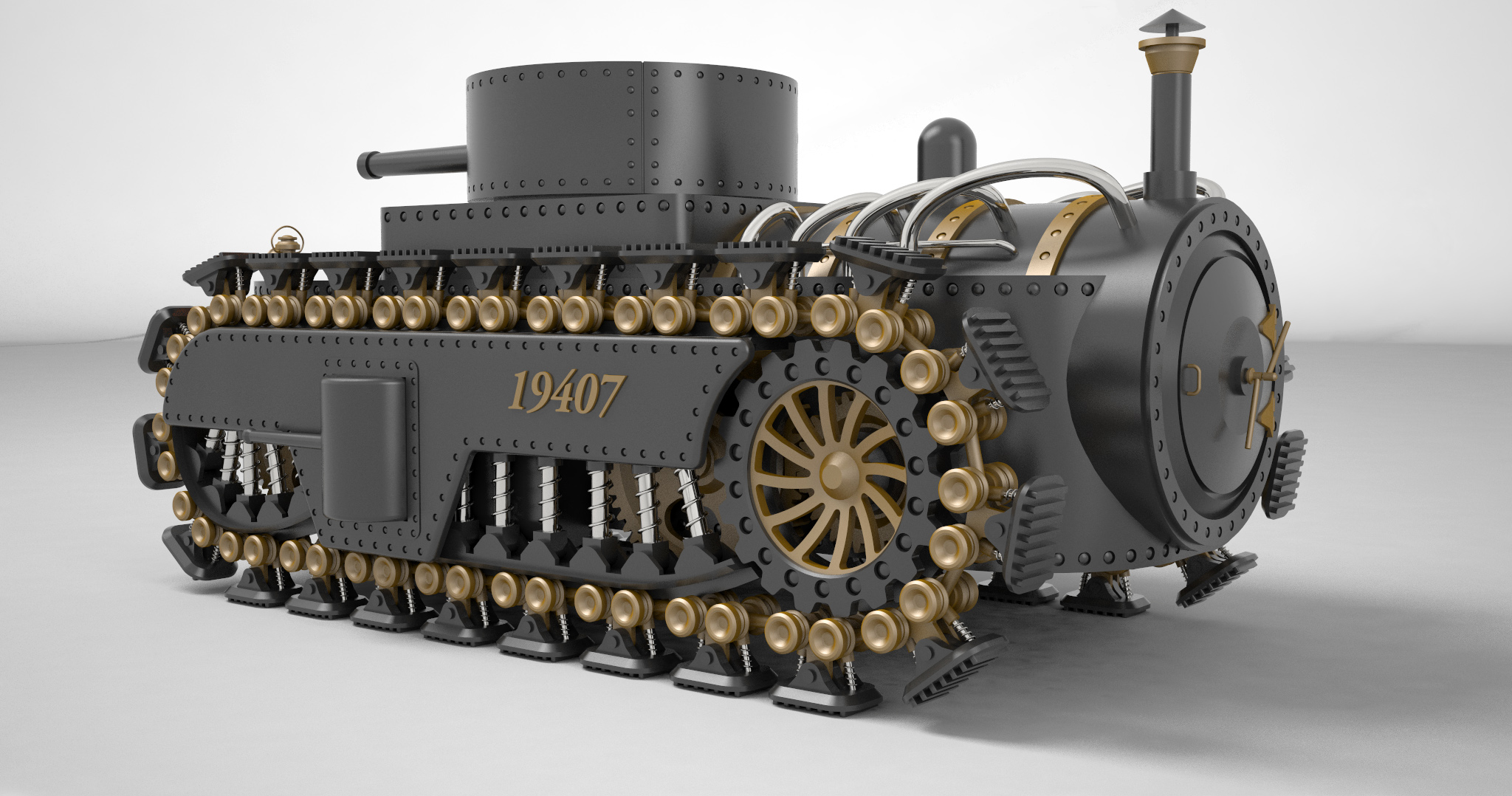The image features a highly detailed, color photograph of a steampunk-inspired, plastic model tank set against a predominantly light gray background accented with darker gray shadows. The tank, centrally positioned and angled as if moving right, showcases a black body highlighted with gold detailing. Prominent steampunk elements include a front cap resembling a locomotive style, a steam pipe above it, and a turret on top with a rifle pointed backward. The tread system features gripper pads and a distinctive gold chain reminiscent of a bicycle chain, linked to sprocket-style wheels. Gold accents also adorn a fan at the front, the top of the whistle, and a front spindle. The side of the tank prominently displays the number "1947" in gold, enhancing its intricate and imaginative design.